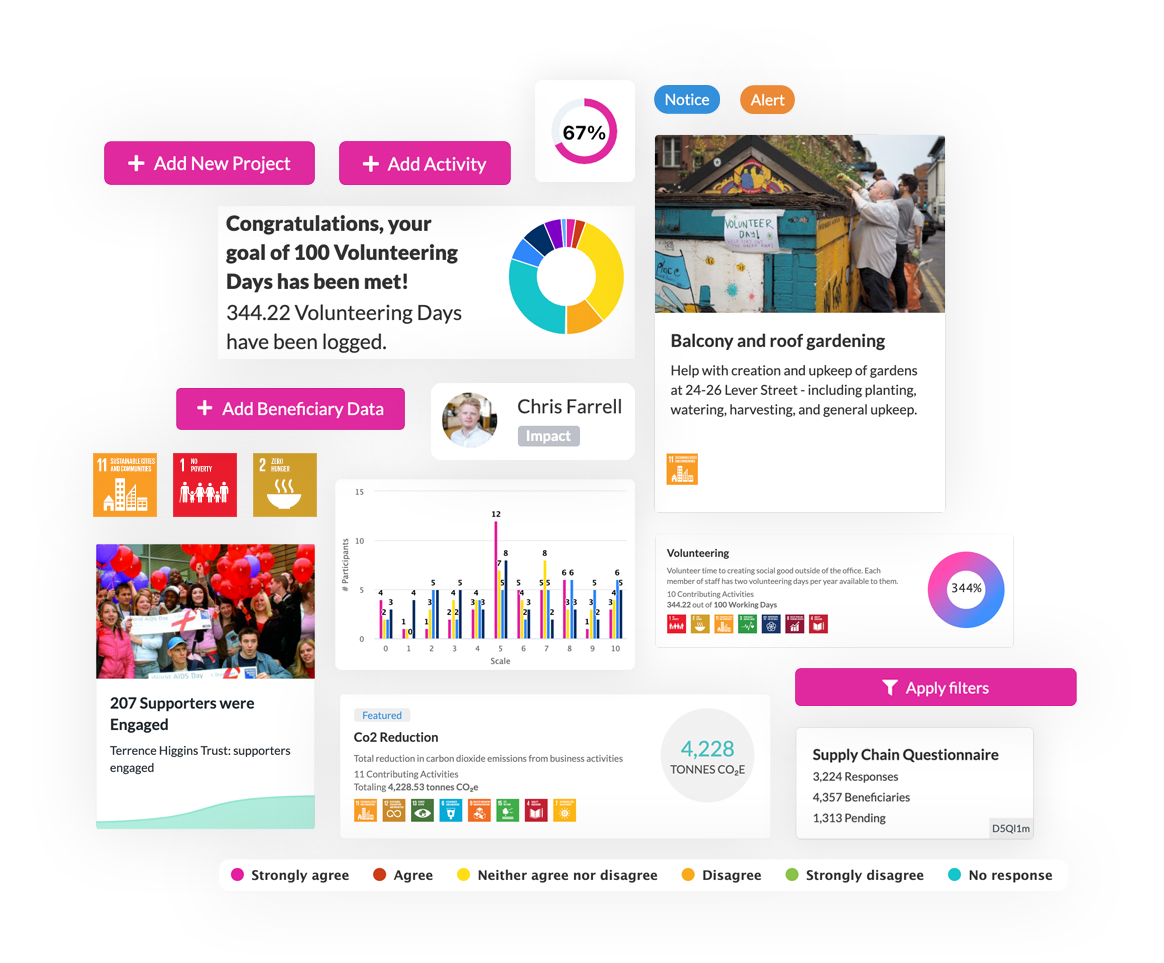This vibrant and detailed screenshot showcases various interactive and informative elements set against a colorful backdrop. At the top of the screen, there are two prominent rectangular buttons in hot pink with white lettering. The first button reads "Add New Project," while the second one says "Add Activity." Adjacent to these buttons is a square displaying the battery percentage at 67%, with the percentage highlighted in hot pink.

To the right of the battery indicator are two small, pill-shaped buttons. The blue button is labeled "Notice" in white letters, and the orange button says "Alert," also in white letters. Below these elements is a vivid photograph depicting several men working on what appears to be a small, colorful shed. The shed is adorned with green and yellow panels, and the men are focusing on fixing the roof. The structure is not very tall, as the men are able to stand while working on it. One man, who appears older and slightly heavyset, is dressed in a white long-sleeve shirt and black pants. Another man, middle-aged, tall, and thin with dark hair, is wearing a gray t-shirt and black pants. The shed is situated outdoors, seemingly in the middle of a road, and there are other indistinct figures in the background.

The caption beneath the photograph reads "Balcony and Roof Garden." To the left of this image, there is a longer rectangular area featuring a colorful circle, likely representing progress or statistics. The circle includes segments in various colors: yellow, orange, green, blue, black, purple, light blue, pink, and red, with the largest sections being yellow and turquoise. Beside this circle, a congratulatory message reads, "Congratulations, your goal of 100 volunteering days has been met, 344.22 volunteering days have been logged."

The page is populated with additional pictures, charts, and tables, contributing to its rich and informative layout.